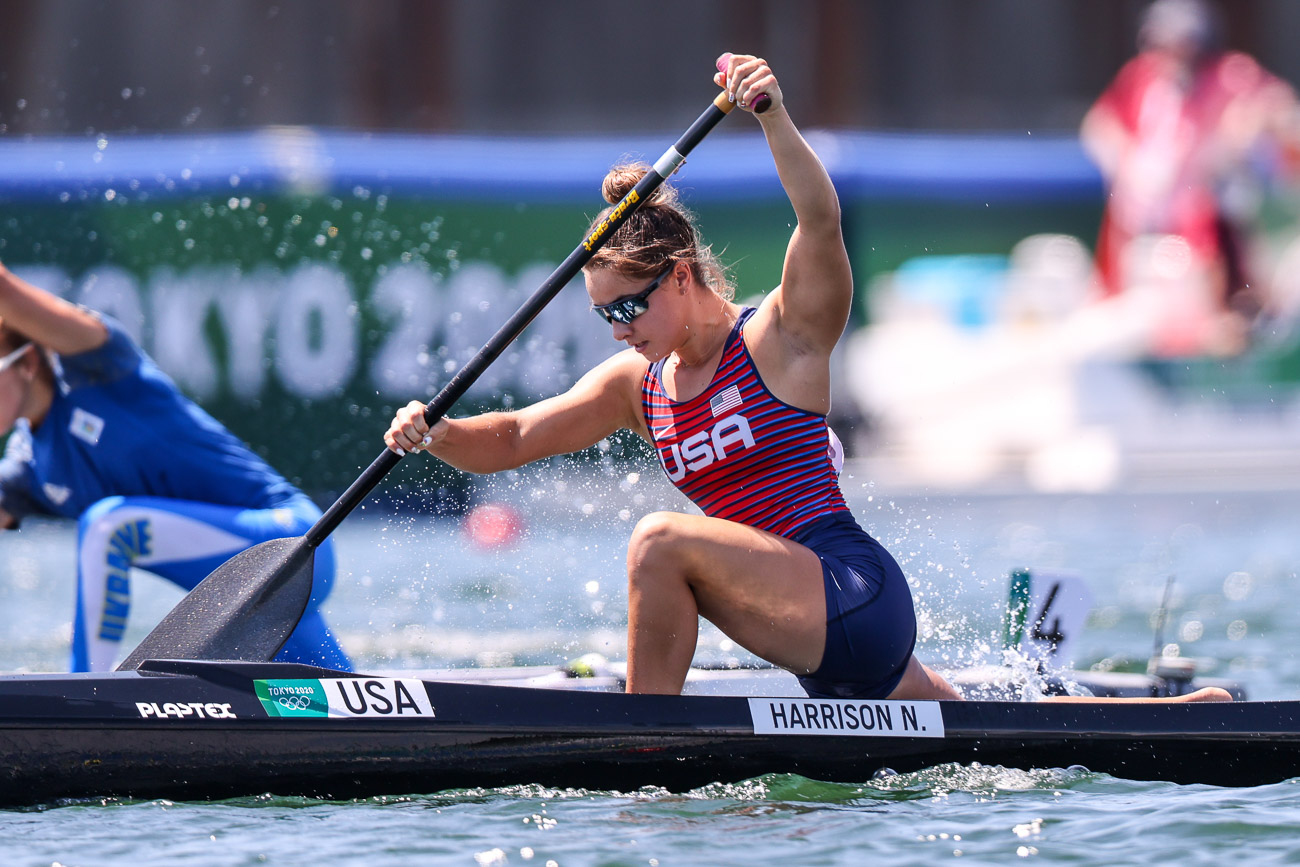The image is a vibrant, action-packed sports photograph from the Tokyo 2020 Olympics, capturing a moment in a major rowing competition. The central figure is a very muscular and focused female athlete, Harrison N., who is firmly gripping her oar as she propels her sleek, black kayak forward through the water. She epitomizes strength and determination, evident in her intense concentration and powerful rowing form. She is adorned in a striking red, white, and blue outfit, a tank top with blue stripes and white 'USA' lettering across her chest, and an American flag emblem near her heart. Her outfit is completed with dark blue shorts, and she shields her eyes from the sun with reflective, dark sunglasses. Visible on her kayak are the black lettering 'USA' and the words 'Tokyo 2020,' indicating the prestigious nature of the event. In the blurred background, another competitor is seen, along with a banner prominently displaying 'Tokyo 2020.' The backdrop is also faintly populated with blurry spectators, adding to the high-stakes atmosphere of this intense Olympic competition.